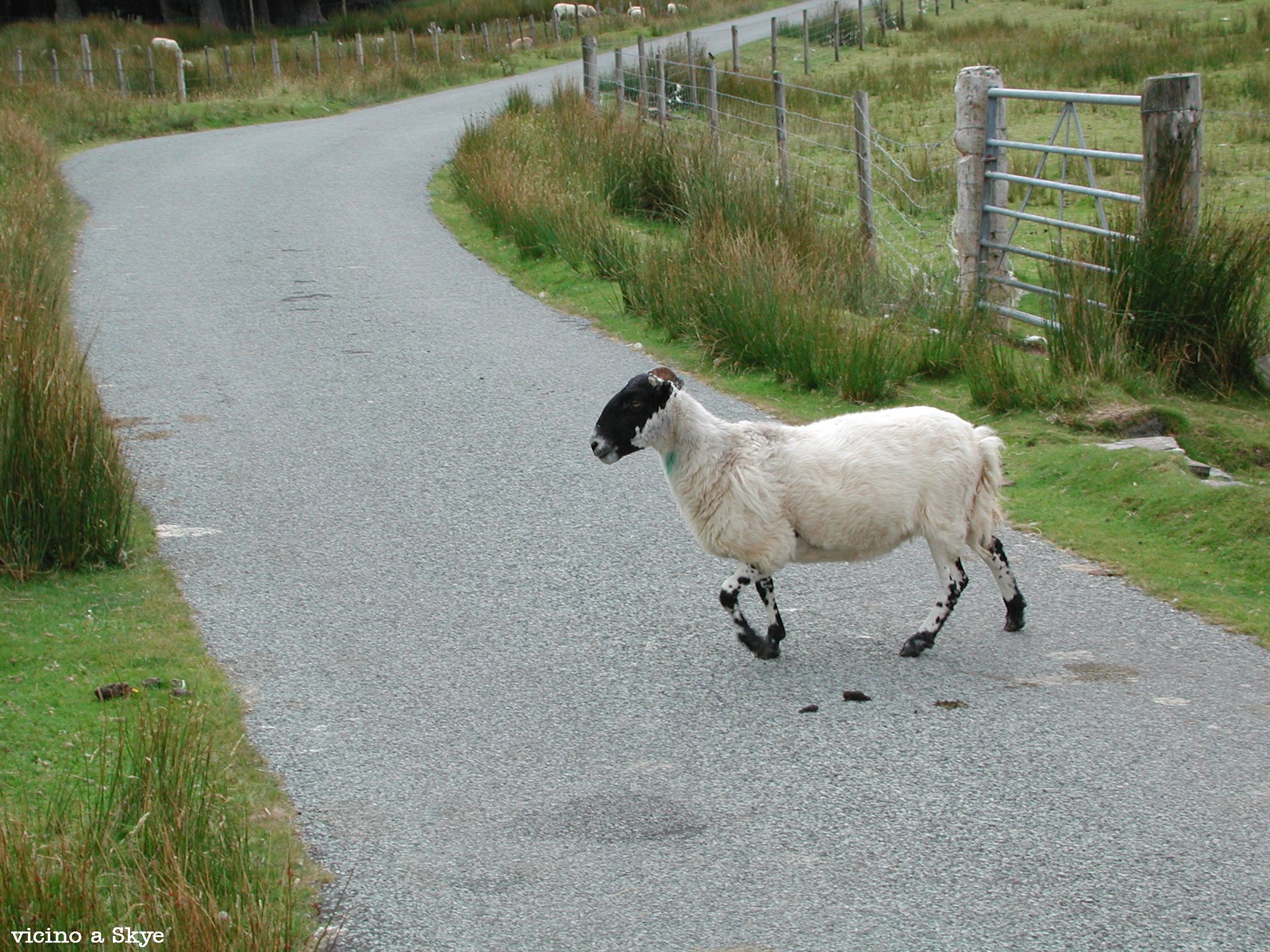This captivating photograph captures a serene countryside scene, featuring a narrow, single-lane paved road curving gracefully from the bottom right to the upper left and back to the center right. Along either side of the gray asphalt road, lush grass and taller reeds sway gently, bordered by rustic wooden posts and wire fencing typical of pastoral landscapes. The focal point of the image is a solitary goat, positioned on the right side, calmly making its way across the road towards a verdant field on the left. The goat stands out with its striking black head, off-white body, and distinctive black and white-spotted hooves. In the distant background, the indistinct silhouettes of more animals—likely goats—add depth and a hint of community to the tranquility of the scene. The only text in the photograph, "Vegino a Skye," is elegantly placed in the bottom left corner. Dominant colors in this bucolic tableau include shades of black, white, off-white, gray, brown, silver, and green, creating a harmonious palette that enhances its timeless, rural charm.